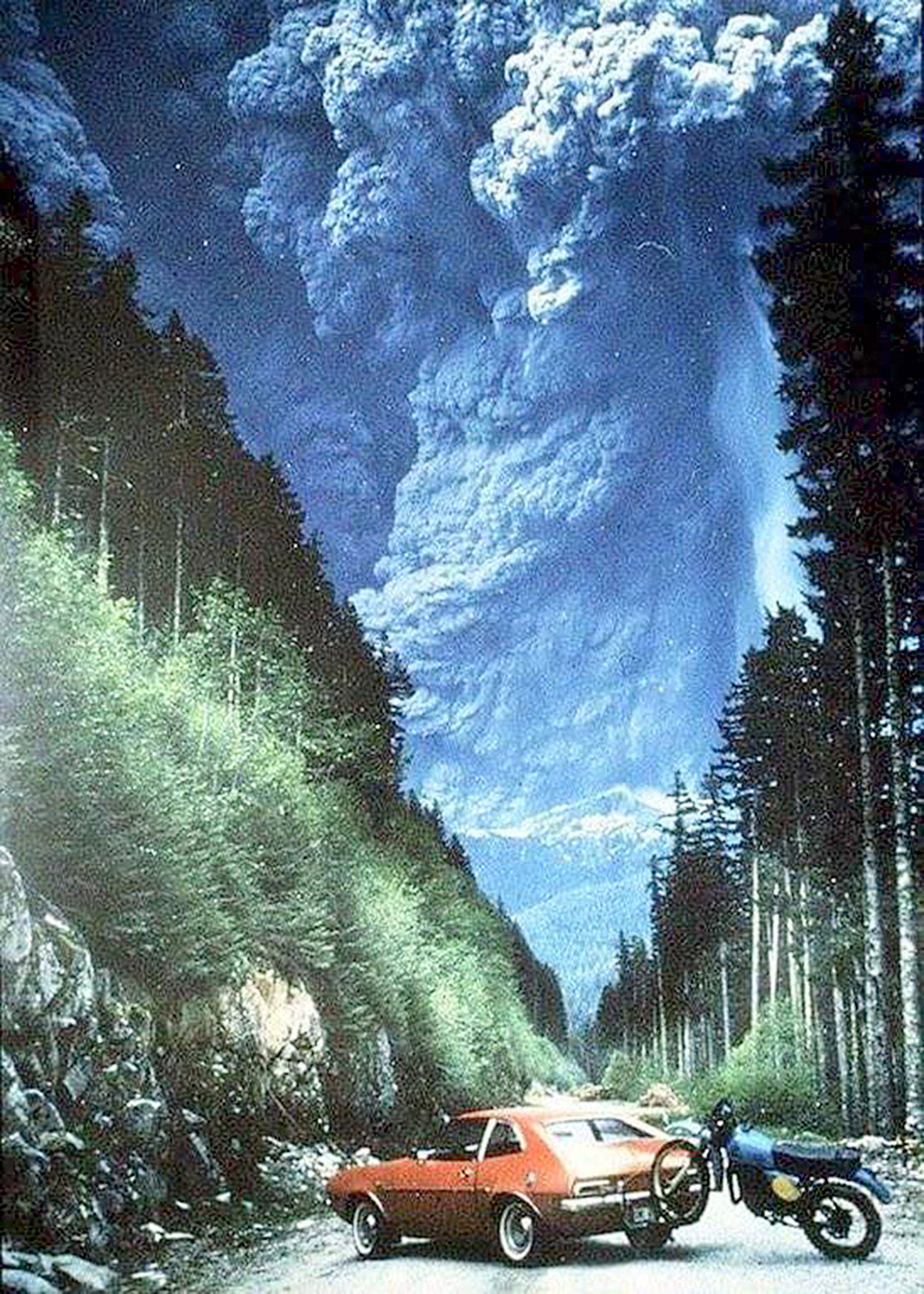The full-color photograph, likely taken in the 1970s during the Mount St. Helens eruption, captures an outdoor scene dominated by a colossal, dark gray cloud of ash and smoke looming ominously above a landscape. The photo is vertically oriented and shows a red car skewed sideways across the road, with a motorcycle tied to its back, seemingly used for towing. No people are visible in the image. The scene is framed by tall, green trees lined on both sides of the road, with patches of grass and rocks scattered around. The backdrop includes faint outlines of mountains shrouded in heavy ash and smoke, creating an overwhelming sense of an impending natural disaster. The suffocating cloud of volcanic ash towers over the scene, dwarfing the vehicles and landscape beneath it with its immense and foreboding presence.